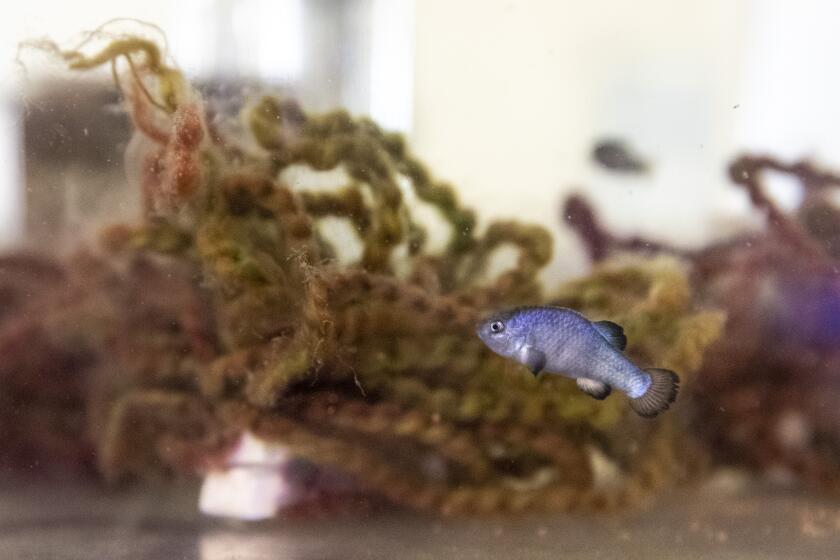In the foreground of this photograph, a fish with a fascinating blend of colors takes center stage. Its body showcases an intricate palette of pale blue, darker blue, gray, and white hues. The fish's tail is an off-grayish color adorned with darker gray frills, adding to its striking appearance. Its single, prominent black eye gazes outward, adding a sense of life and curiosity to the scene.

In the background, a rich tapestry of underwater life unfolds. A verdant green plant provides a lush backdrop on one side, while on the opposite edge, another plant with earthy brown and burgundy tones adds depth and contrast. Further in the distance, another fish can be faintly discerned, partially obscured by the softly blurred background that features an intermingling of tan and white shades. Gentle shafts of sunlight filter through, illuminating the underwater landscape and adding a touch of warmth to the image.